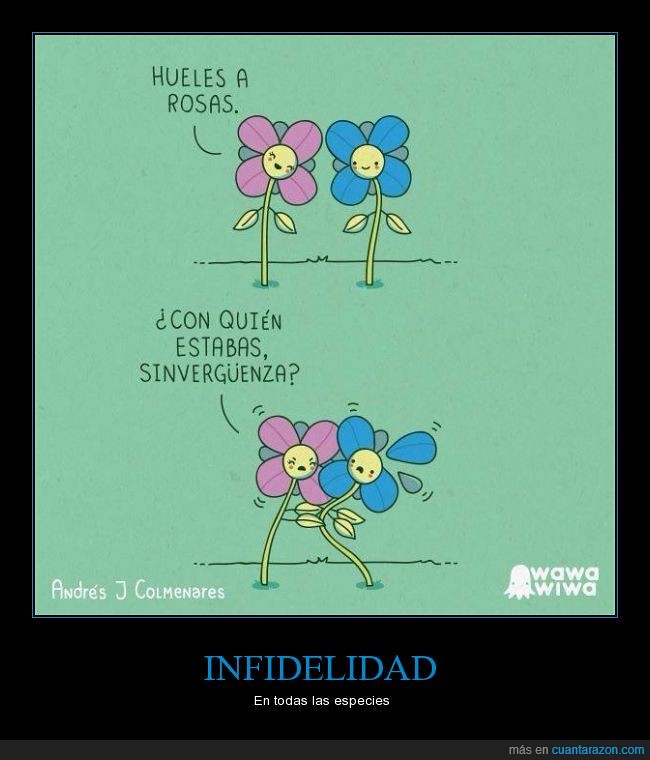The image appears to be a comic-style poster or ad, framed with black edges and a green center. It features two flowers, a pink one and a blue one, depicted in two separate panels. Both flowers have eyes and mouths, adding a personified touch to the scene. In the top panel, the pink flower, standing to the left and resembling a girl, is smiling and speaking to the blue flower, which resembles a boy and stands to the right. The text above the pink flower reads, "Hueles Rosas," which is likely a compliment. The blue flower is responding with a smile. 

In the bottom panel, the mood shifts dramatically. The pink flower appears angry and is using its leaves to shake the blue flower, causing it to lose a petal. The text above the pink flower reads, "¿Con quién estabas, sinvergüenza?" which suggests a confrontation about infidelity. The blue flower looks distressed and bent from the force. 

At the bottom of the poster, in white and blue text, are the phrases, "Infidelidad en todas las especies" (Infidelity in all species), "Andres J. Colmenares," the creator's name, and "Wawa Wiwa" with a small drawing of an octopus. The overall scene conveys a humorous yet dramatic narrative about infidelity among anthropomorphic flowers.